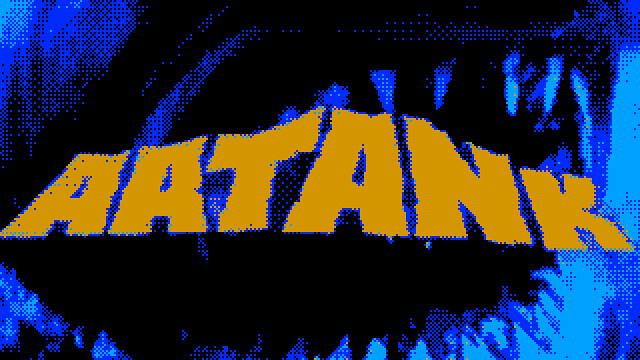This left-to-right horizontal image appears to be a pixelated, computer-generated artwork, possibly sourced from a video game. The background is a mosaic of tiny squares, predominantly in various shades of blue, intermixed with black, giving it a digital, almost retro aesthetic. The sides of the image are primarily blue, while the center features a darker, nearly black section, interspersed with blue shapes resembling jagged teeth descending vertically. At the top, clusters of blue and black pixels create a dotted texture. In the foreground, bold orange letters span from left to right, standing out against the pixelated backdrop. These letters, "AATANK," are styled to appear three-dimensional, with a subtle outline that blends the blue and black dots from the background, enhancing their prominence and depth.